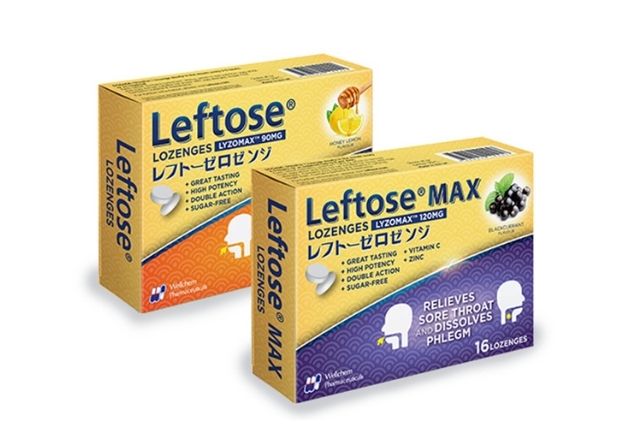The image showcases two retail boxes of Lefto's Max Lozenges, designed to relieve sore throats and dissolve phlegm. The boxes are arranged with one in front of the other, slightly angled to expose most of the text on the rear box. Both boxes share a beige upper half, while their lower halves differ in color and flavor indication—orange for the orange-flavored lozenges and purple for grape-flavored lozenges. Each package contains 16 lozenges and features vibrant colors including yellow, orange, and purple. Both boxes display a combination of English text and Asian characters, emphasizing the product's high potency, sugar-free, vitamin C with zinc formula. Additional highlights include phrases like "Great Tasting" and "Double Action." The packaging also displays images of the respective fruits and a graphic depicting a lozenge being placed into a mouth. The setting suggests a medical environment, possibly implying endorsement by medical staff for phlegm relief.